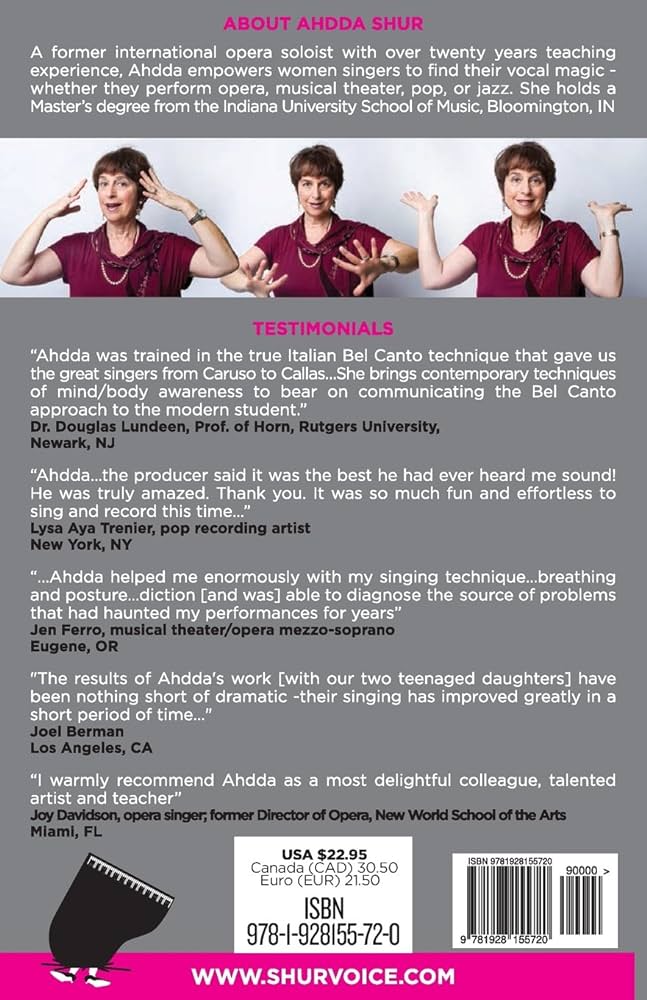This appears to be the back cover of a book focused on Ada Shure, a former international opera soloist with over 20 years of teaching experience. Ada holds a master's degree from the Indiana University School of Music, Bloomington, Indiana, and is dedicated to empowering women singers across various genres such as opera, musical theater, pop, and jazz.

The top portion of the back cover features three photographs of Ada, a middle-aged woman with short brown hair, dressed in a dark red short-sleeved blouse, and wearing what seems to be a pearl necklace. In the photos, she is posed differently: one with her hands on either side of her head, another with her hands pressing outward, and the last one with her hands in a shrugging gesture.

Following the photographs, a series of testimonials highlight Ada's expertise. Dr. Douglas Lundin, a professor of horn at Rutgers University, praises her mastery of the Italian bel canto technique and her integration of modern mind-body awareness practices. Lisa Aya Trenier, a pop recording artist from New York, shares that her producer considered it her best performance, attributing it to Ada's effective teaching methods. Jen Farrow, a mezzo-soprano in musical theater and opera, attributes her improved singing technique, breathing, posture, and diction to Ada's guidance. Joel Berman from Los Angeles notes dramatic improvements in his teenage daughters' singing abilities. Lastly, Joy Davidson, an opera singer and former director of opera at the New World School of the Arts in Miami, Florida, commends Ada as a delightful colleague and talented artist.

The back cover also includes essential details such as a barcode and ISBN code, pricing information for the USA (22.95 USD), Canada (30.50 CAD), and Europe (21.50 EUR), and a quirky black cartoon of a piano crushing someone with feet sticking out. At the very bottom, a hot pink strip provides Ada Shure's website: www.shurevoice.com.